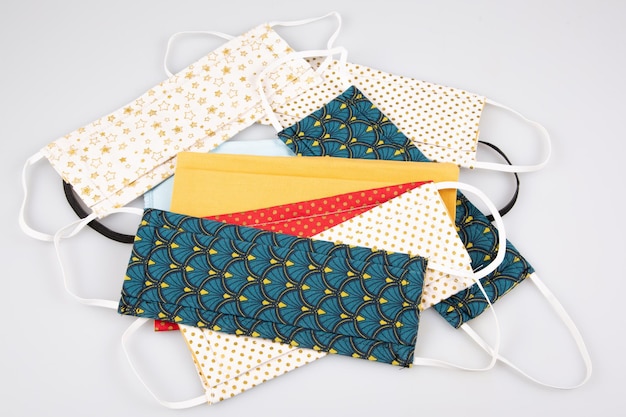The image features a central pile of six fabric face masks, commonly used during the COVID-19 pandemic. Each mask showcases a unique design and pattern, with some sharing similarities. Among the masks, two exhibit dark blue backgrounds adorned with gold and black fan-shaped designs. Another two masks share a white base, densely covered with orange stars. Additionally, there is one mask that is entirely orange and another one that pairs red and orange hues. A mask with a yellow background and small yellow geometric prints is also present. The masks, haphazardly overlaid upon one another, highlight their varied styles against a plain white backdrop, with visible ear attachments indicating their functionality.